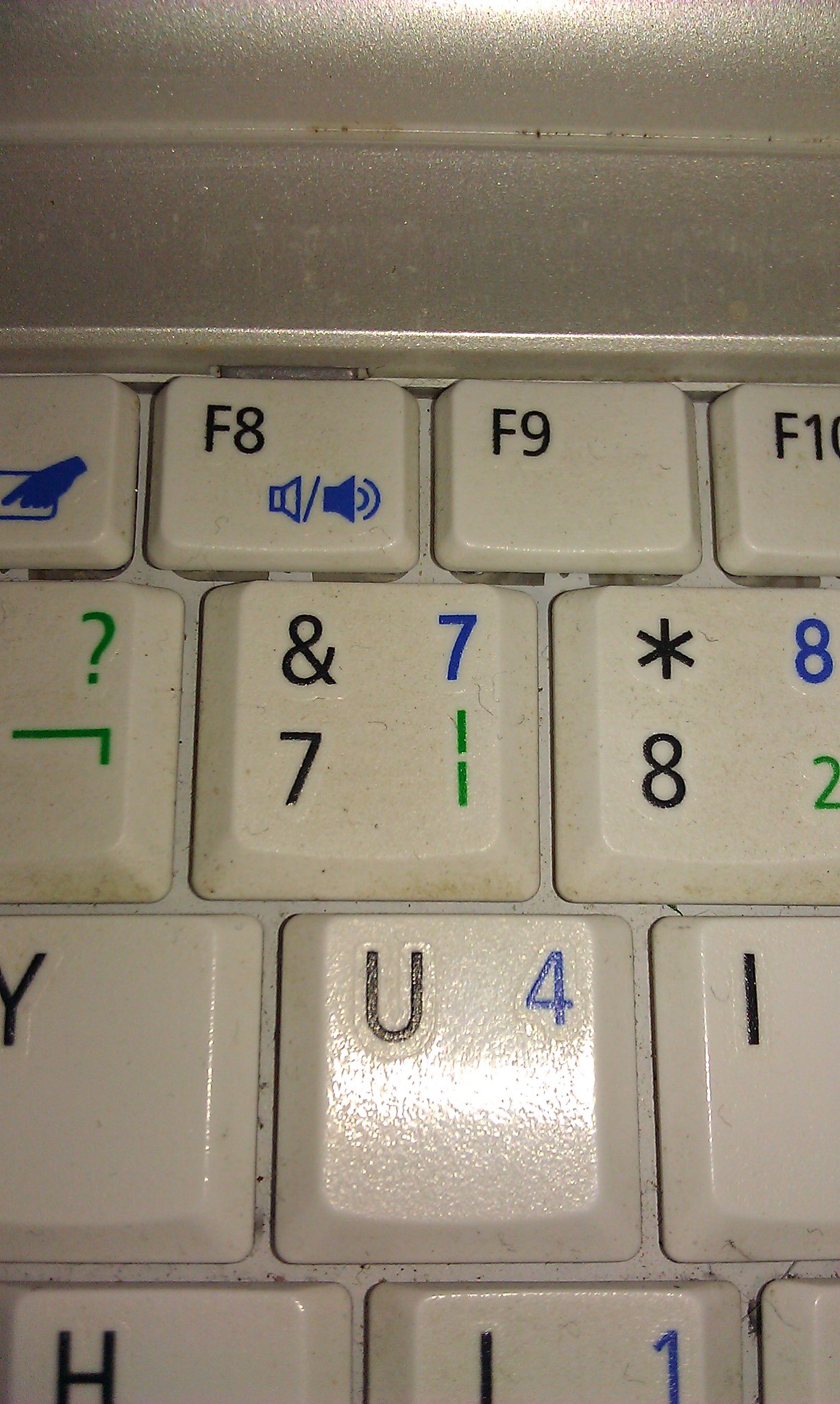This photograph captures a close-up section of a light beige computer keyboard, focusing on a few specific keys. At the top, the image showcases the F8 and F9 function keys, with the F8 key featuring volume control icons. Below these function keys are the number keys: 7, which includes an ampersand symbol when shifted, and 8, which has a vertical bar symbol. These keys exhibit a mix of black, green, and blue markings. Further down, the entire U key is visible, flanked by the partially visible Y and I keys, which extend out of the frame. The keys display varying symbols and functions, creating a colorful and detailed snapshot of this section of the keyboard.